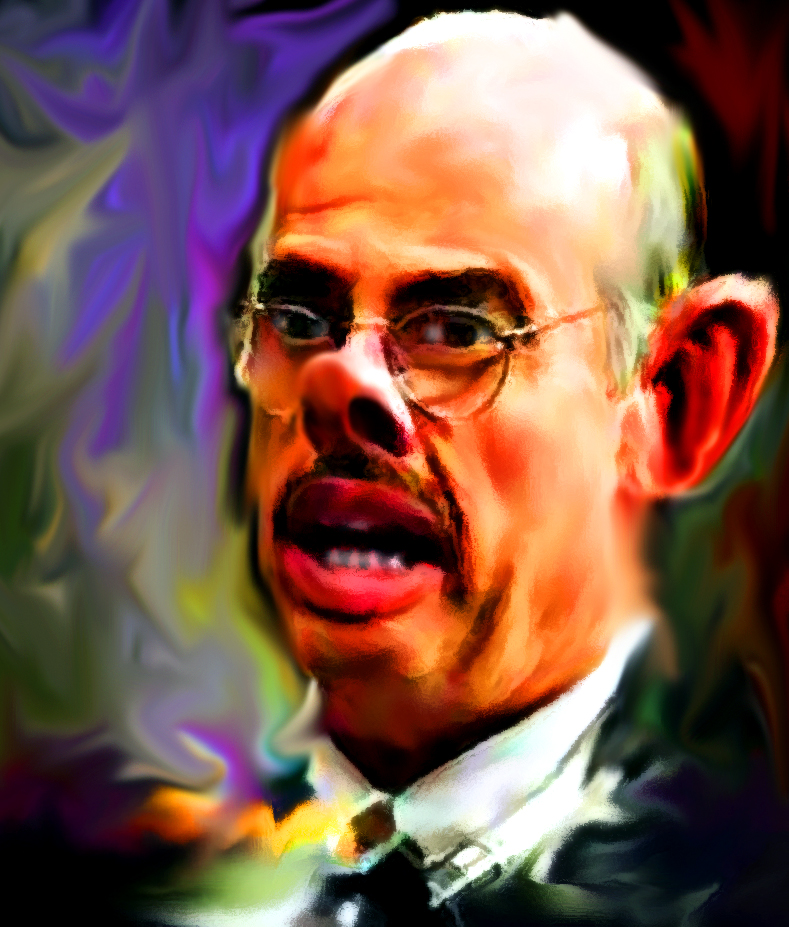This is a digitally created painting of a bald, white male political figure or possibly a judge, characterized by a distinctive and unflattering exaggerated depiction. The subject wears wire-rim glasses, a white shirt, and a dark suit jacket. The painting emphasizes his large pig-like nose, oversized ears, thick lips, and thick eyebrows, contributing to a distorted, almost grotesque appearance. The background is filled with swirling textures in chaotic hues of purple, green, yellow, red, and black, intensifying the sense of turmoil and frantic energy in the composition. Despite its digital nature, the artwork mimics traditional brushstrokes and manages to be both colorful and highly embellished, presenting a vivid, albeit unkind, representation of the man.